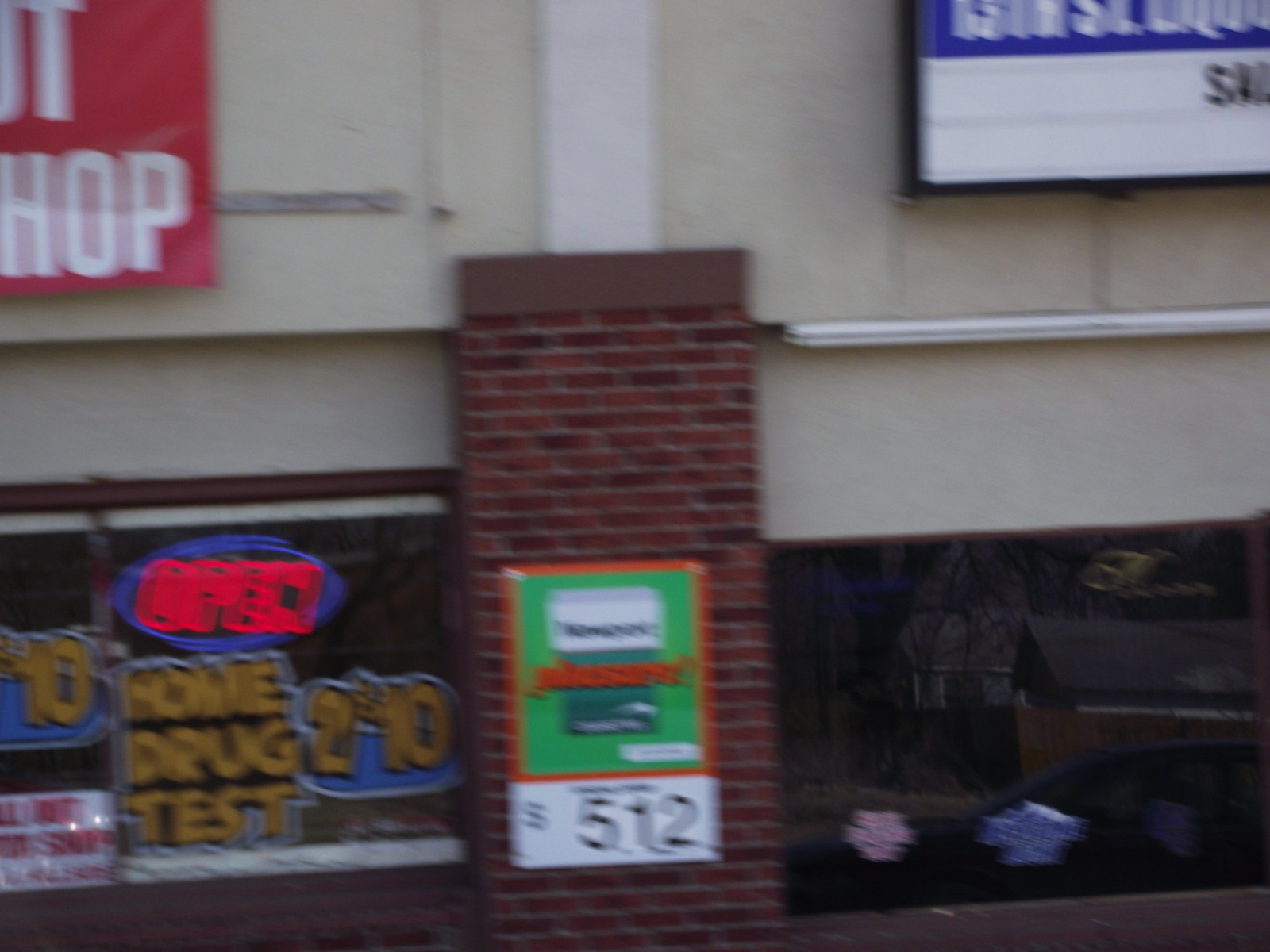In this photograph, a series of storefronts are displayed, creating an eclectic and visually interesting urban scene. The facade prominently features a tan-colored wall, punctuated by a section of red brick that runs vertically down the center. This brick portion hosts an advertisement for Newport cigarettes, showcasing a white and green package with "Newport" written in bold letters. Below, in orange print, the word "pleasure" is visible, along with a boxed price tag stating "$5.12" in white.

To the right side of the image, a black window storefront reflects a fence line, a car, and a building situated across the street, adding layers to the scene. On the left, a vibrant neon sign reading "open" in red is encircled by a blue outline, signaling the store's readiness to welcome customers. Adjacent to this, yellow text on a black background advertises "home drug test two for $10", catering to practical consumer needs. A partially visible sign on the far left, also in yellow, mentions a "$10 off" discount, though it's slightly cut off from view, adding to the fragmented yet comprehensive snapshot of urban commerce.